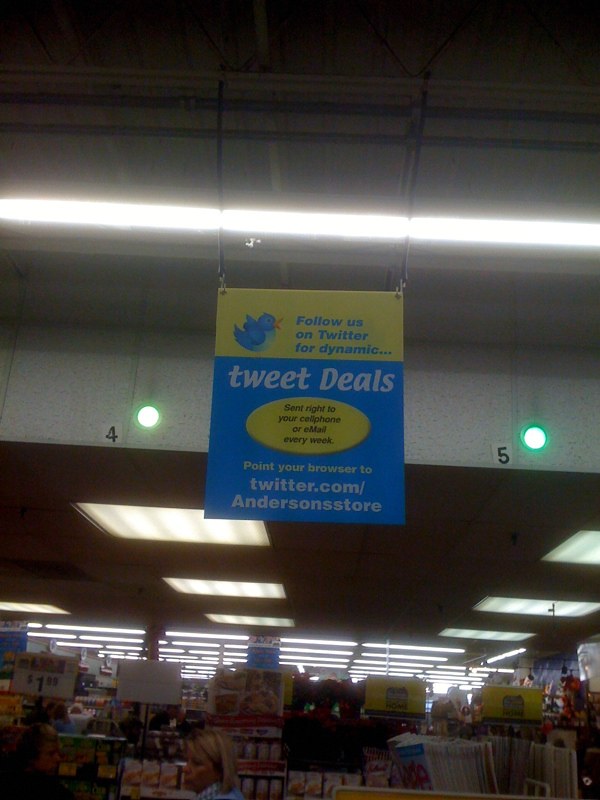The image captures the interior of a grocery store, prominently featuring a detailed banner hanging from the ceiling by corded wires. The store's high ceiling, painted gray with exposed black piping, is adorned with long, rectangular fluorescent lights. The shelves below are stocked with an assorted mix of items, including rolls of toilet paper, boxes of food, books, and magazines. People move through the aisles beneath the sign, giving a lively atmosphere. 

The banner itself is rectangular with a yellow top and a blue bottom. The top portion reads "Follow us on Twitter for dynamic..." in blue font, accompanied by a small blue Twitter bird logo. Beneath this, the blue section displays the phrase "Tweet Deals" with "Tweet" in lowercase and "Deals" starting with a capital "D". In the center of the banner, a yellow lozenge-shaped oval contains the message, "Sent right to your cell phone or email every week," with the word "email" notably styled with a lowercase "e" and an uppercase "M". 

Directly below this, the banner instructs viewers in yellow font to "Point your browser to," followed by "twitter.com/AndersonStore" in white font. Adjacent to the banner, the ceiling features small green lights labeled with the numbers 4 and 5, further illuminating the store below.